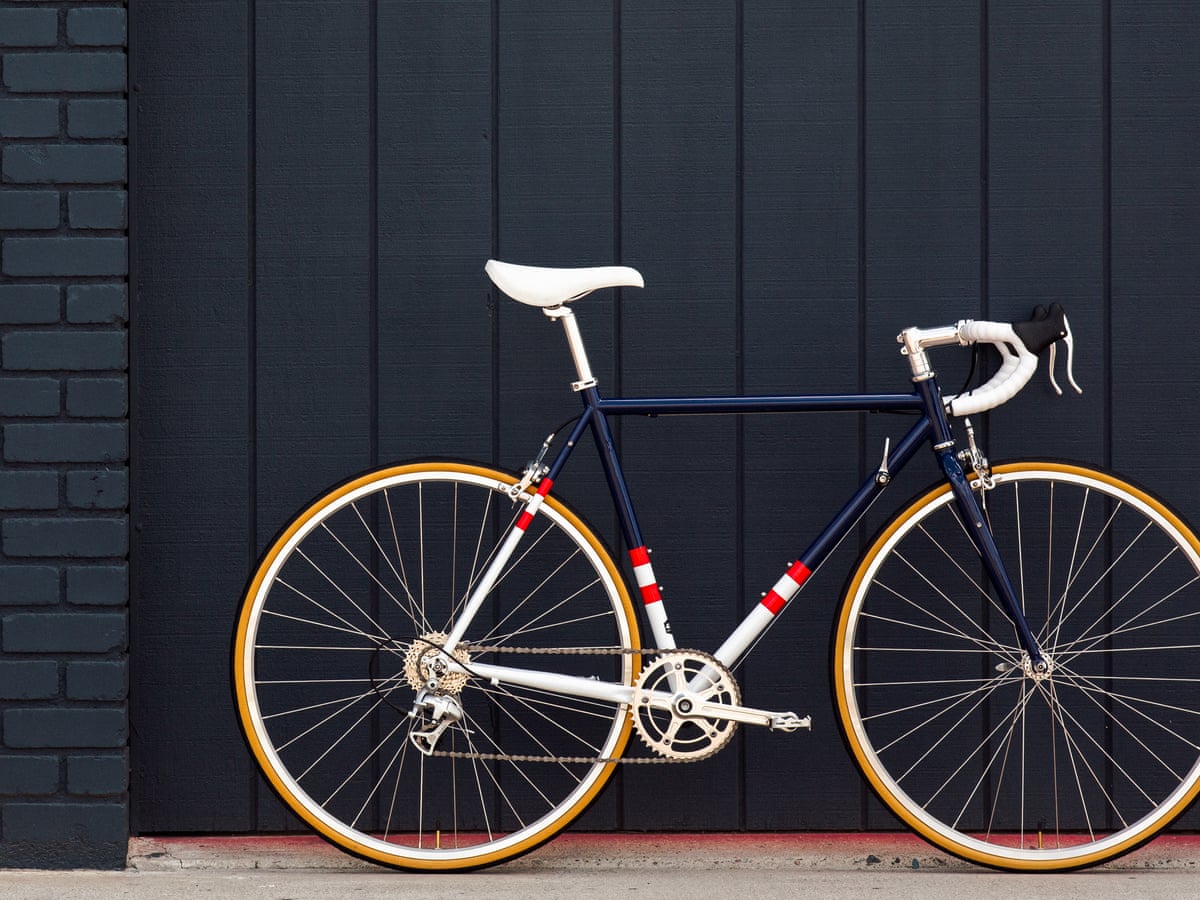The color photograph features a side view of a bicycle positioned against a dark blue, paneled wooden wall, resembling part of a gate. To the left of the image is a column of dark blue brick wall. The bicycle’s frame is predominantly navy blue, transitioning to a white section adorned with red rings near the bottom of the triangular frame and around the chain area. It has distinctive white handlebars with black ends and a matching white seat. The large wheels of the bicycle feature an orange outer rim, although some describe them with yellow coloration with white lines. The ground beneath the bicycle is gray pavement. The blue paneled wall includes a gray baseboard with a pink stripe above it. The bicycle is oriented to the right of the image in this plain and simple composition, devoid of any writing, people, animals, or motorized vehicles.